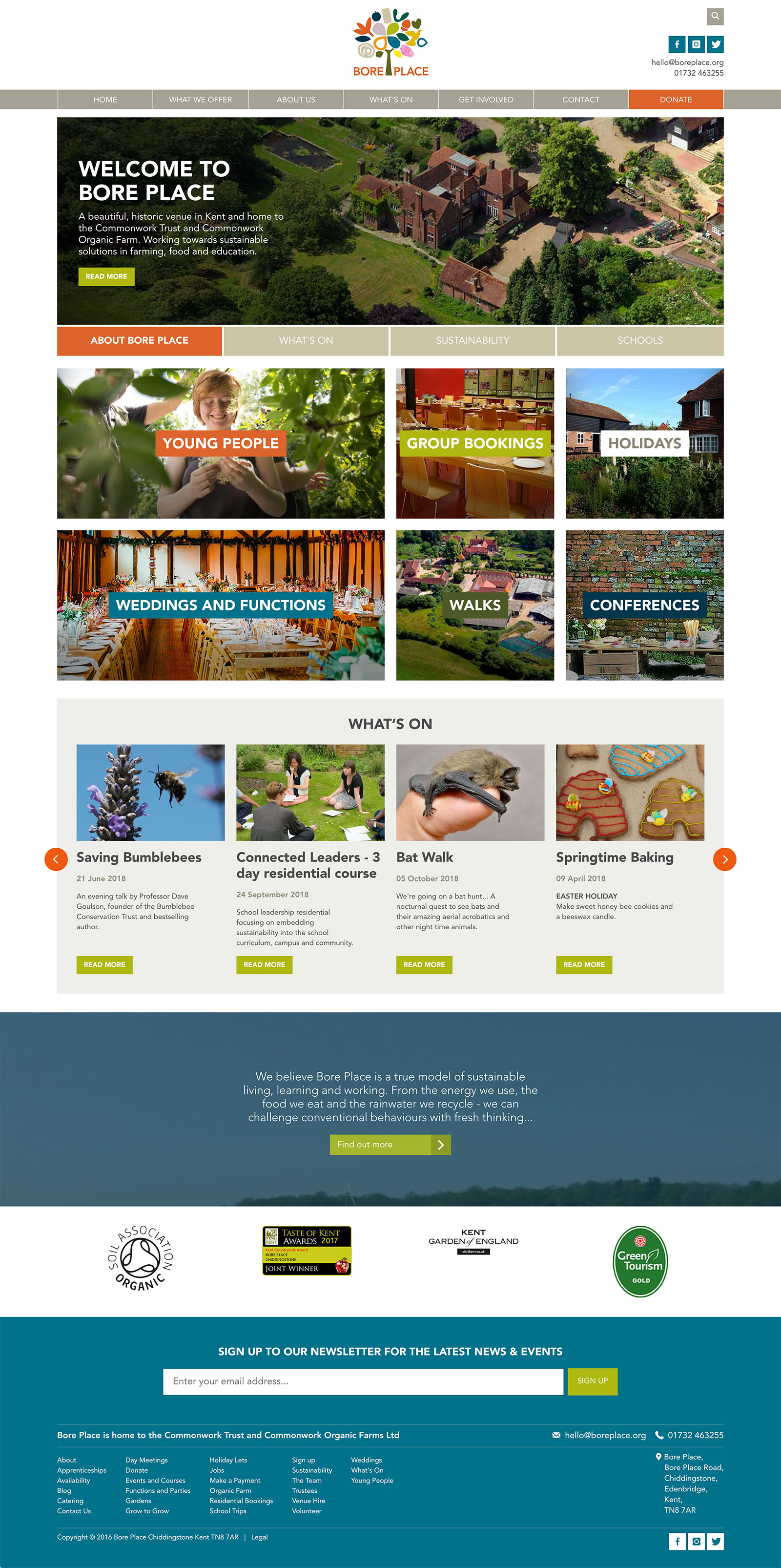The image depicts a desktop version of a website viewed on a mobile device, resulting in a cluttered and hard-to-read layout. At the top of the screen is the logo of "Boar Place," featuring a colorful tree. Directly below the logo is some text that is too small to decipher. The main banner prominently displays an image of a grand castle or large historic house surrounded by beautiful gardens. This suggests that Boar Place is a historic estate open to the public, possibly functioning as a museum or a site where visitors can pay for tours and explore the grounds.

Beneath the banner, there are various navigation links including "About Boar Place," "Young People," "Group Bookings," "Holidays," "Weddings and Functions," "Walks," and "Conferences." These indicate the range of activities and services offered at the estate. Additional sections include articles on topics related to the estate and its surroundings, such as one about saving bumblebees and another detailing a bat walk, highlighting the site's commitment to environmental and educational initiatives.